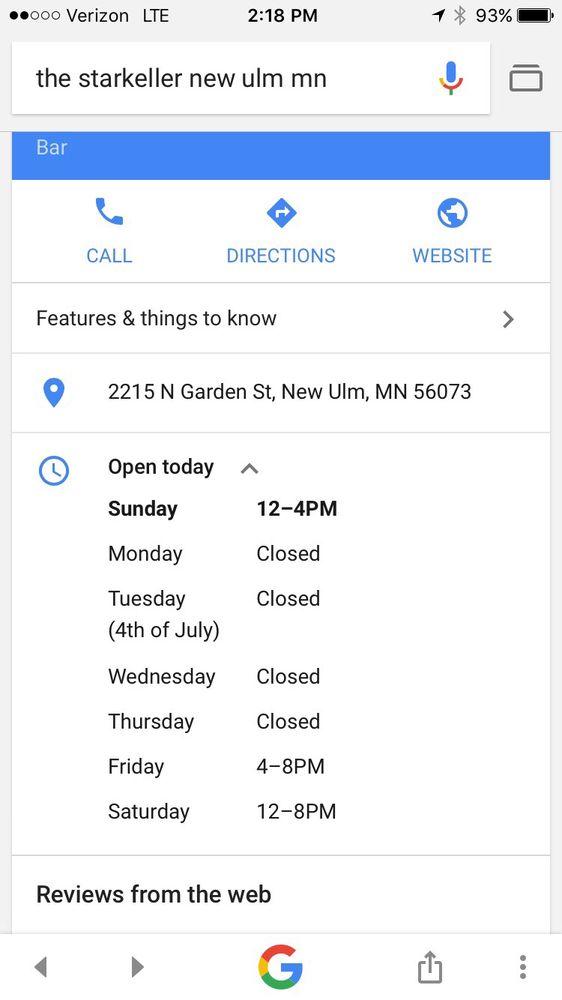The computer screen displays a variety of information and options. At the very top, the labels show "Verizon LTE" on the left, the current time "2:18 PM" in the center, and a battery level of "93%" on the far right. Beneath this status bar, the screen features a location header that reads "The Starkeller, New Ulm, MN". Below this, a microphone icon is visible, followed by a prominent blue bar labeled "Bar" in white text.

Further down, three interactive icons are displayed: 
1. "Call" with a phone image,
2. "Directions" featuring a white arrow within a blue diamond,
3. "Website" indicated by a globe icon.

Under these icons, there's a section titled "Features and Things to Know," marked by a black arrow pointing to the right. The address "2215 North Garden Street, New Ulm, MN 56073" is listed below this heading.

The operating hours are specified as follows:
- Open today, Sunday: 12 to 4 PM,
- Monday: Closed,
- Tuesday: Closed (4th of July),
- Wednesday: Closed,
- Thursday: Closed,
- Friday: 4 to 8 PM,
- Saturday: 12 to 8 PM.

Next, a row titled "Reviews from the Web" appears, accompanied by navigation arrows; a gray arrow points left, and another faces right. In the center of this section is the Google "G" icon, signifying reviews sourced from Google.